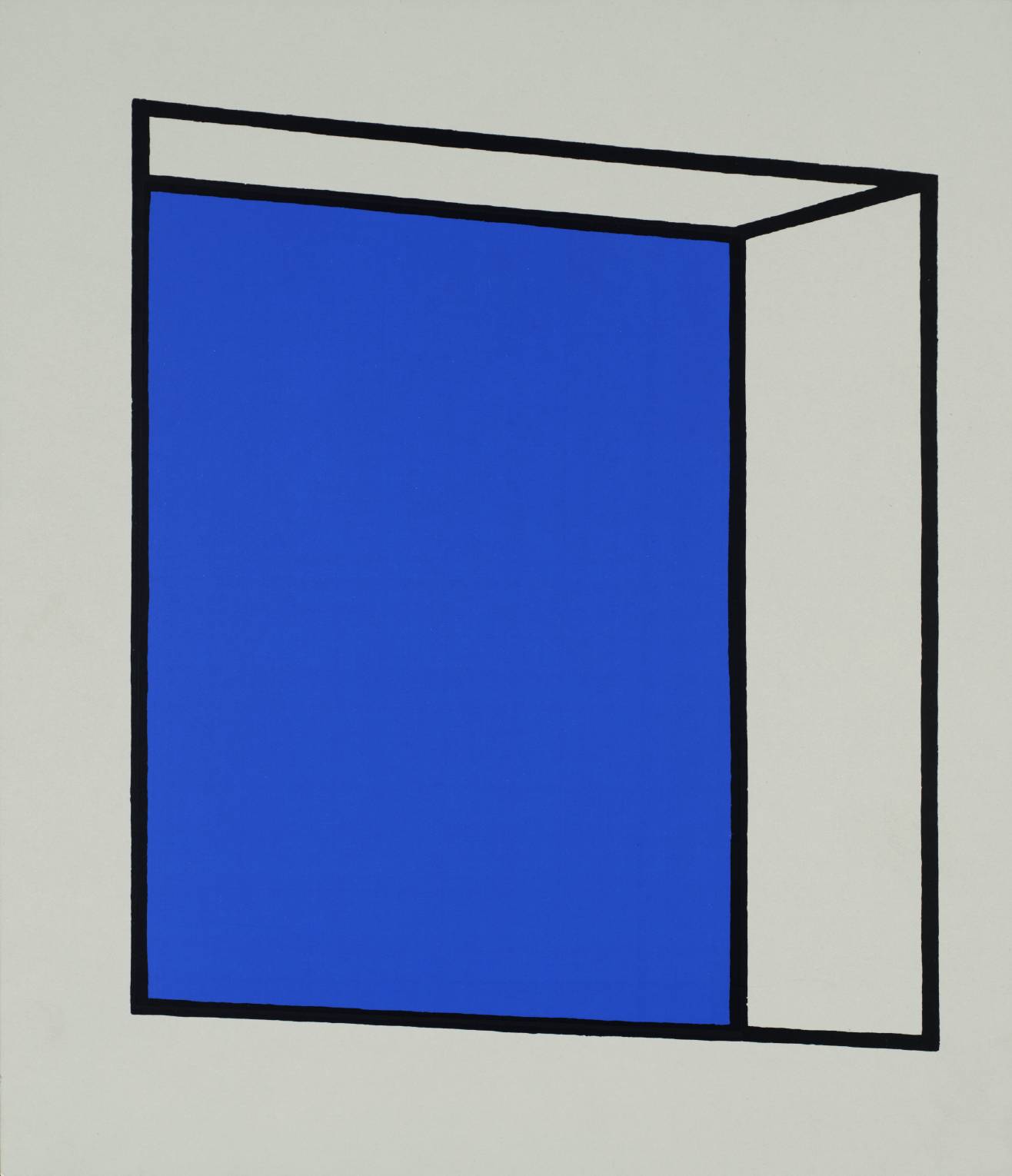This is a simplistic yet striking color graphic design titled "Small Window" by artist Patrick Caulfield, created in 1969. The artwork features a minimalistic composition set against a light gray background, with the central figure being a vividly blue rectangle outlined in bold black lines. The blue rectangle, symbolizing a window, is complemented by two attached gray rectangles—one extending to the right and one on top, together forming an abstract, stylized outline of a book or window. The window, portrayed in a stark white surrounding, offers a view of a perfectly blue sky, reminiscent of the blue and white aesthetics seen in Santorini, Greece. This piece, rendered in a photorealism, modern art style, captures a clean and refined essence, employing simple geometric shapes to create a sense of depth and perspective.